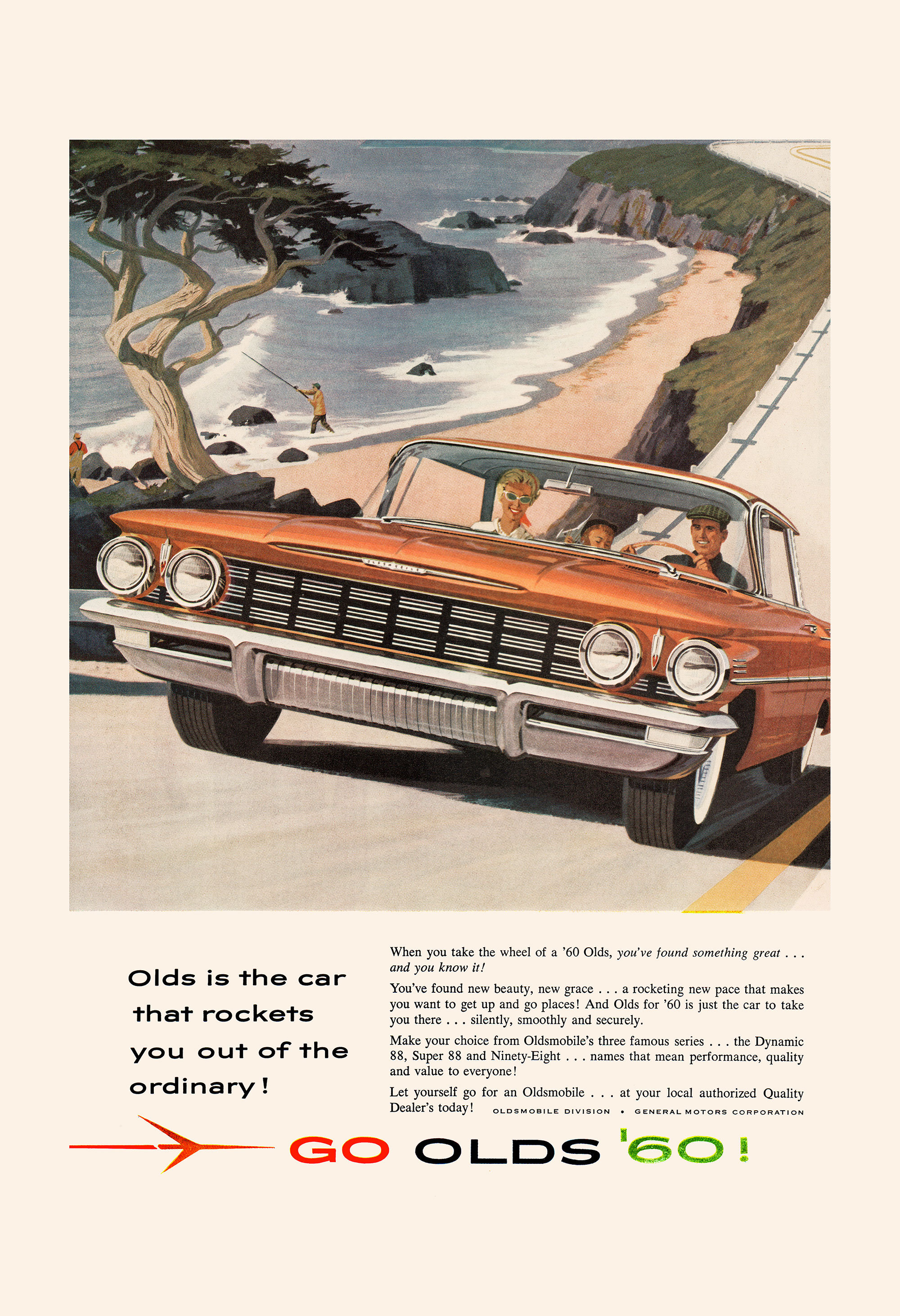This vintage 1960s advertisement features an idyllic coastal scene, centered within a square-cropped magazine layout. The background is an off-white color and showcases a picturesque highway running along the edge of a cliff, framed by waves crashing against dark gray rocks and a windswept pine tree. On the water below, a fisherman in a yellow coat and black pants casts his line into the surf.

Dominating the scene is a bright orange, boxy Oldsmobile, driving slightly uphill and almost towards the viewer. The car, indicative of the 1960s style, boasts four headlights, a metallic white bumper, and a wide grille. Inside, a smiling man in an old-fashioned driving cap grips the wheel, while his wife, donning chic white sunglasses and a fashionable white blouse, sits beside him. Though mostly obscured by the dashboard, their child peeks over from the back seat.

Beneath the image, vivid text declares, "Olds is the car that rockets you out of the ordinary." Further details extol the virtues of the car, highlighting its new beauty, grace, and a rocketing pace that invites adventure. The advert emphasizes the reliability and quality of Oldsmobile’s three famous series: the Dynamic 88, Super 88, and 98. It concludes with a compelling call to action: "Let yourself go for an Oldsmobile, at your local authorized quality dealers today," signed off by the Oldsmobile Division of General Motors Corporation. Accompanying this text is a striking logo featuring a thin, thorned rose branch in red, alongside "Go Olds 60!" with the word "Go" in red, "Olds" in black, and "60!" in green.